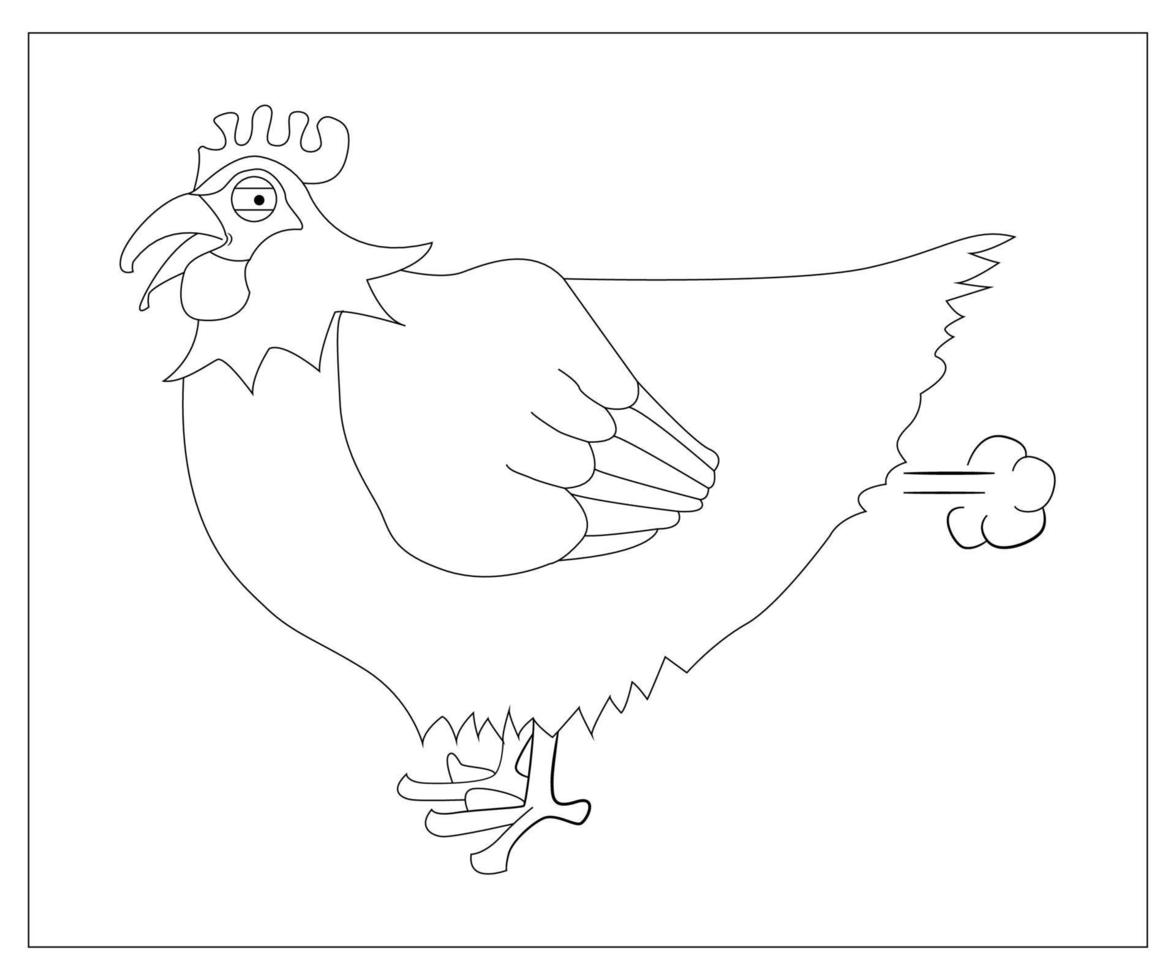This is a black-and-white line drawing of a caricatured rooster, facing to the left and depicted in a side view. The illustration, rendered in either pen or dark pencil, features exaggerated proportions with notable elements including a curved beak, a lidded eye, and a distinctive comb composed of four ovals on top of its head. The rooster sports a feathered stomach, a large wing with variable thickness, and small, disproportionate feet. Additionally, it has feathers extending off its head and a rounded detail under its beak. A humorous touch is added with a small cloud or puff of smoke emanating from its rear end, suggesting it is passing gas. The drawing is set against a plain white background and enclosed within a thin black box. The simplicity of the drawing contrasts sharply with its whimsical subject matter, making it an amusing and detailed piece.